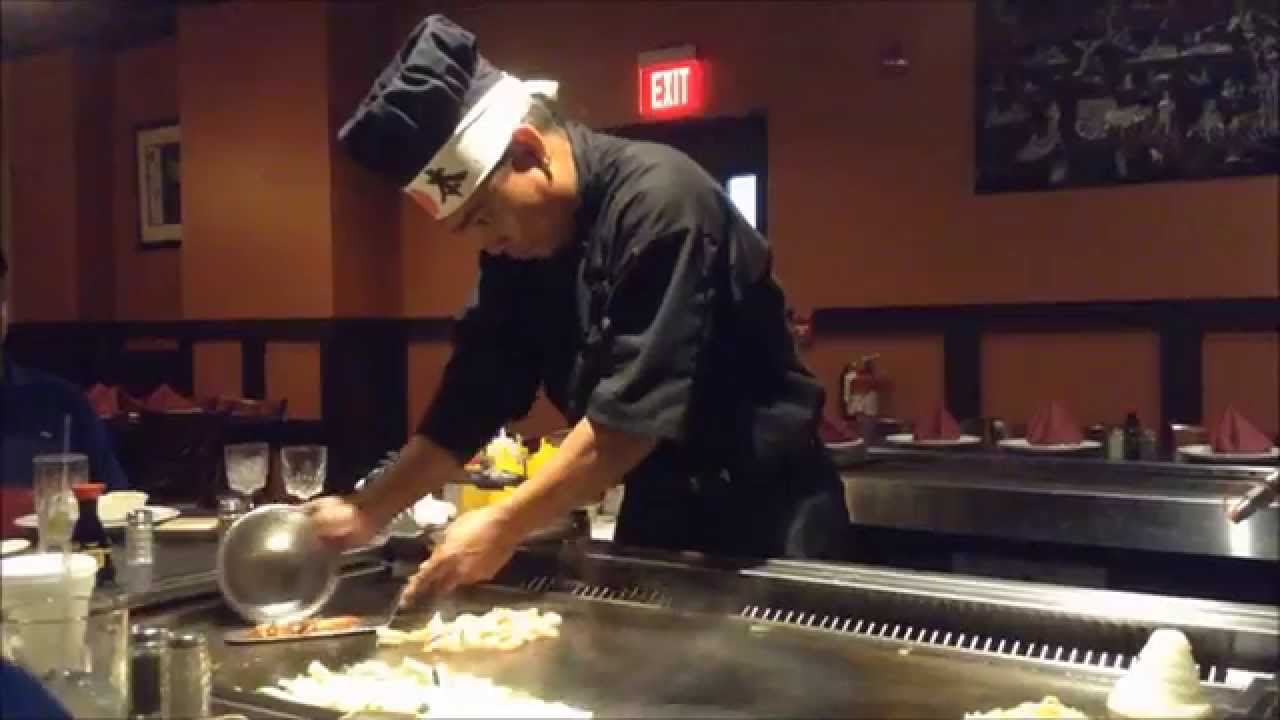This is a photograph of a Japanese hibachi chef, possibly an Asian man, deeply focused on his culinary craft. The chef is dressed in a black uniform consisting of a black shirt, apron, and hat, complemented by a white bandana adorned with kanji letters. He is seen at a grey-colored workstation, actively mixing food items in a vessel. Surrounding him are several glasses, bowls, and plates with red napkins, suggesting he is in the midst of preparing a meal. The background features a dark orange wall with brown paneling, a grey rectangular wall art, and a brightly glowing exit sign with white font on a red background. Behind him also stands a grey countertop extending the visually cohesive setup. The overall setting exudes a restaurant ambiance, hinting at a busy yet orderly environment expected in a hibachi dining experience.